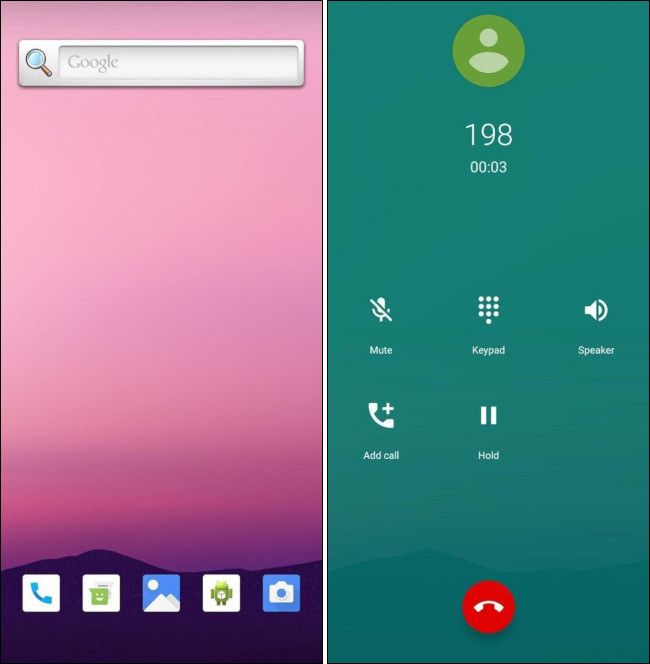The image displays two screens from a tablet or cell phone. 

The left screen features a serene backdrop with a captivating purple-to-pink gradient. The sky transitions from light pink at the top to a deep purple near the bottom, evoking the ambiance of twilight. Silhouetted against this gradient is a simplistic, purple-hued mountain range, adding a touch of natural beauty. At the top of this screen is a Google search bar. Along the bottom, there are five app icons in a row: a phone icon for dialing, a green speech bubble with a smiley face representing messages, an icon for the gallery app, a symbol of the Android mascot, and a camera icon.

The right screen shows the device in use during an active call. The same mountain range image is visible but now features a turquoise blue overlay for differentiation. The call interface displays prominently, offering buttons for mute, keypad, speaker, add call, and hold options. A call has been ongoing for three seconds with the number '198' shown. At the bottom of this screen, there is a red button to end the call.